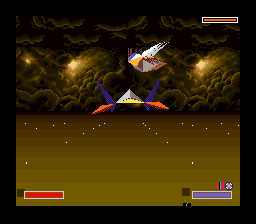This screenshot from a video game showcases a vibrant, multi-layered green field under a sky filled with peculiar spacecraft. Two distinct crafts hover above the landscape: the first is a silver triangle with a yellow lower deck, featuring blue and orange accents, while the second, positioned higher, is a similarly colored silver and yellow craft with additional blue highlights. The backdrop is adorned with ethereal green clouds illuminated by yellow lights, enhancing the otherworldly atmosphere. On the game's HUD, a red bar appears in the bottom left corner, and a purple-lavender colored bar is present in the bottom right corner, likely indicating player statistics or in-game elements.